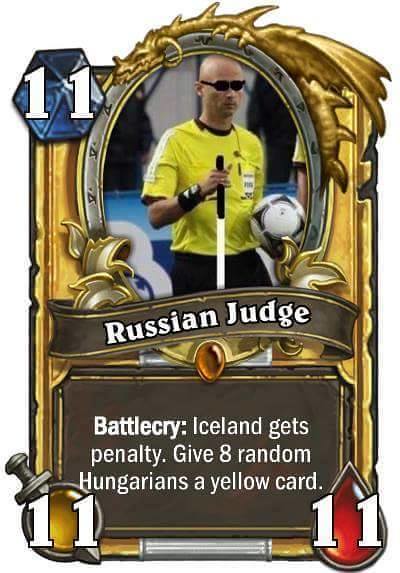The image resembles a decorative playing card, framed in an intricate gold design with accents of dragons and swords. In the center is a silver, oval-shaped portrait of a bald man wearing black sunglasses and a yellow soccer jersey, holding a cane in one hand and a soccer ball in the other. Above the oval, a gold dragon is wrapped around it. The card features several jewels: a large blue jewel on the left, a yellow jewel pierced by a dagger also on the left, and a teardrop-shaped red jewel on the right, all with the number 11 printed in white. Below the portrait, a banner reads "Russian judge," and beneath that, in a rectangle, it says "Battle Cry: Iceland gets penalty, give eight random Hungarians a yellow card." The overall design and layout evoke the style of a collectible card game, with detailed art and imaginative elements.